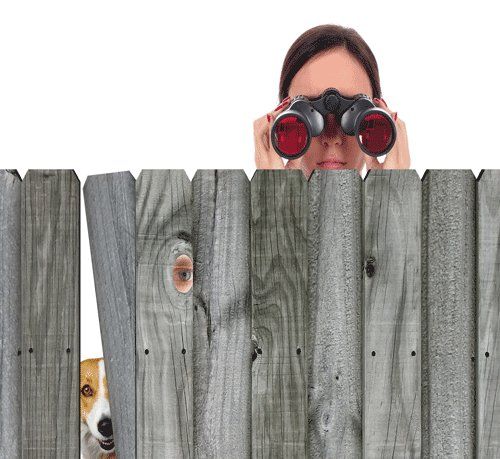In this intriguing photograph, a weathered gray wooden fence dominates the scene. The fence, made up of slats with visible knots and dark nails, features a peculiar triangular gap where one board has tilted slightly. Through this gap, a beige and white dog peeks, revealing one expressive eye. Adjacent to this, a small knothole exposes a single human eye, blue-gray with a hint of green. Above the fence, a white woman with dark brown hair peers through a pair of binoculars with striking red lenses, her nails painted a matching red. The background remains starkly white, devoid of any trees or grass, keeping the focus entirely on the intriguing figures obscured yet visible through the fence.